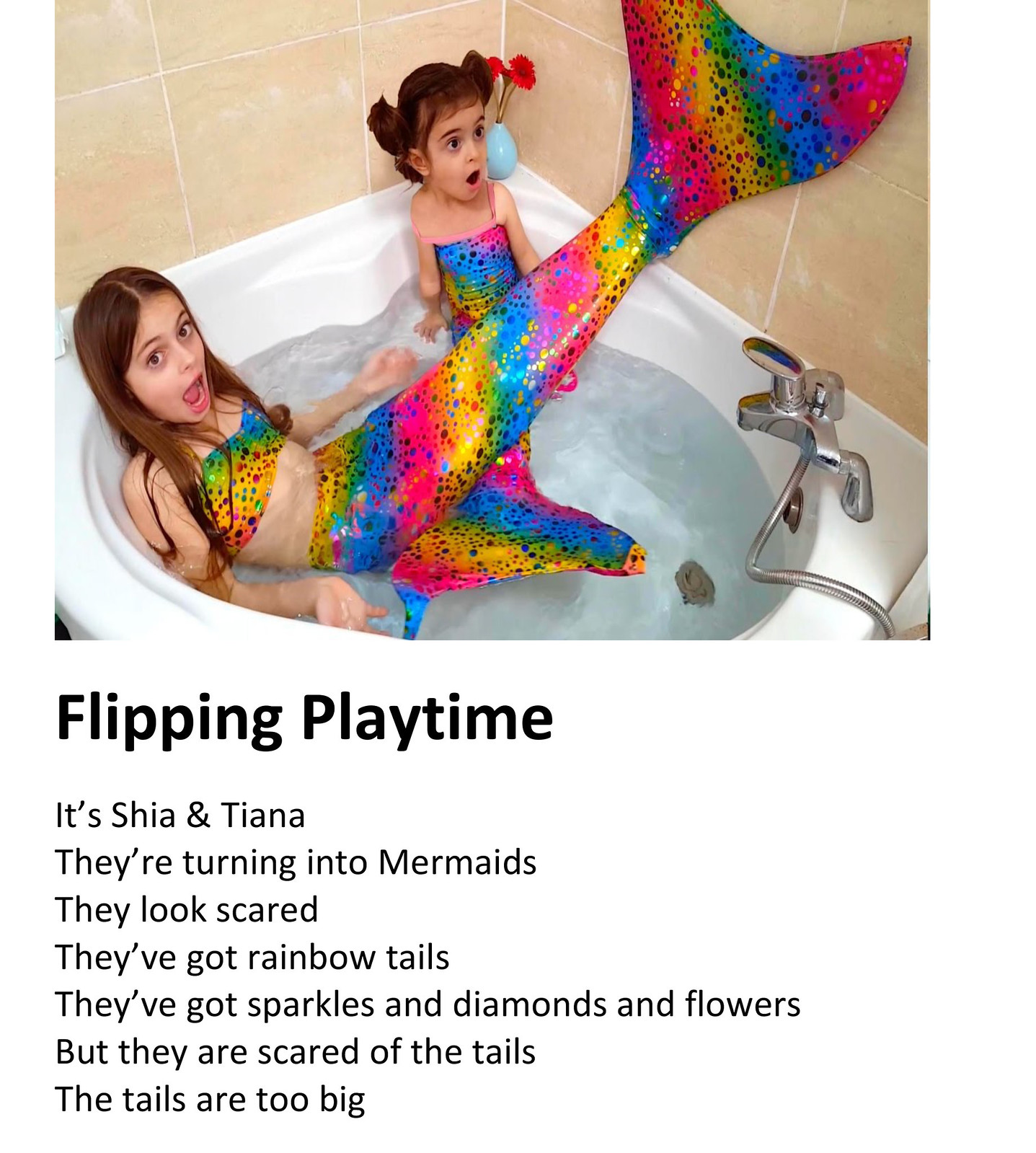This vibrant and whimsical photograph captures two young girls, Shia and Tiana, immersed in a playful yet startling transformation into mermaids within a large, water-filled bathtub. The older girl, approximately seven or eight years old, is dressed in an elaborate, rainbow-colored mermaid outfit adorned with sparkles, diamonds, and flowers. She gazes directly at the camera with her mouth agape and eyes wide open, clearly surprised. Her younger sister, around three or four years old, also dons a similar, smaller mermaid ensemble and is looking off to her left. Both girls exhibit expressions of shock and apprehension, seemingly intimidated by the overwhelming size of their mermaid tails. The bathtub, which is round and filled to the brim with water, is set against a backdrop of large, camel-colored tiles. The image is captioned "Flipping Playtime" in bold black text, followed by the line, "It's Shia and Tiana. They're turning into mermaids. They look scared. They've got rainbow tails. They've got sparkles and diamonds and flowers, but they are scared of the tails. The tails are too big."